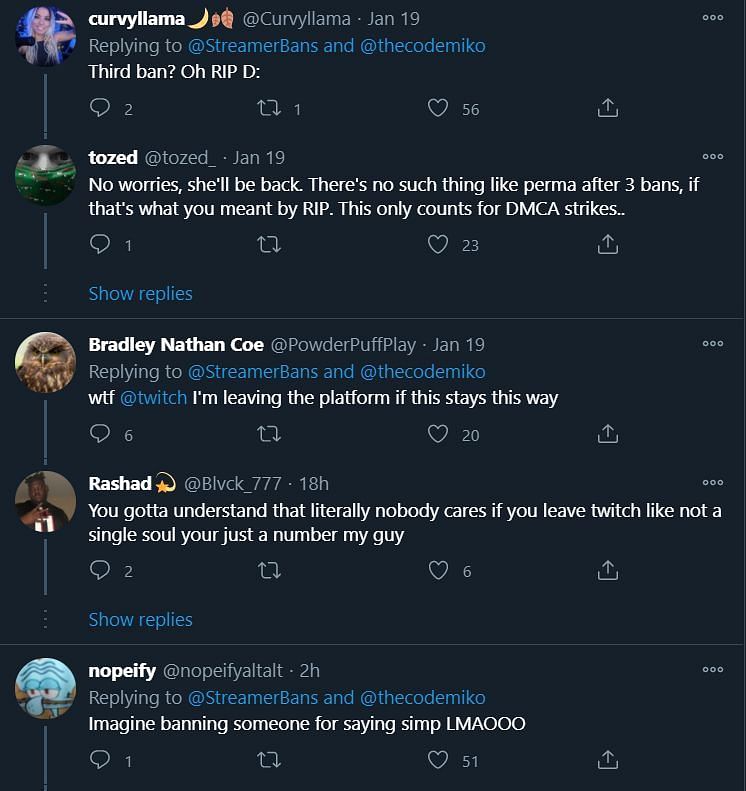This image is a screenshot of a Twitter (now X) conversation regarding the platform's banning policies, displayed in dark mode. The main thread begins with a tweet from Curvy Llama replying to streamer bands and Code Miko, stating, "3rd ban, RIP 😢," which has garnered 56 likes, 2 replies, and 1 retweet.

Following this, Toast responds reassuringly, "No worries, she'll be back. No such thing as permanent after three bans if that's what you meant by RIP. This only counts for DMCA strikes." This tweet invites more responses hidden behind a "show replies" button.

Bradley Nathan Cole from Powderpuff Play then chimes in, replying to streamer bands and Code Miko with, "WTF @Twitch Omni, the platform if it stays this way," which receives 20 likes and 6 replies. Rashad counters Bradley's comment, saying, "You gotta understand that literally nobody cares if you leave Twitch; not a single soul. You’re just a number, my guy," securing 6 likes and 2 replies.

One of the subsequent replies is from Notepify, addressing streamer bands and Code Miko. They mock, "Imagine banning someone for saying simp lmaoo," which resonates with the users, earning 51 likes and one reply.

The dark mode setting features a black background, and each user's profile picture is clearly visible beside their responses, adding a personal touch to the online discussion.